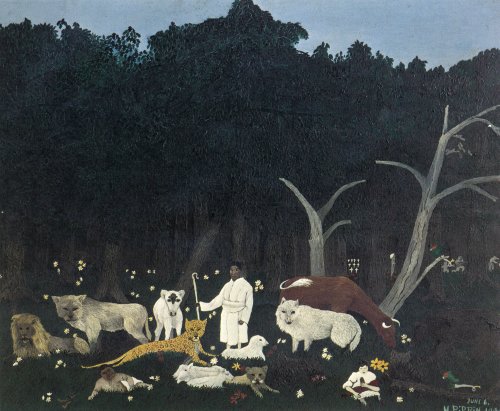In this detailed painting, a young African man dressed in a white shepherd's robe stands at the center, holding a shepherd's staff with a hook. Surrounding him is an array of animals: a lion with a mane reclining to his left beside a standing lioness, a cheetah lying at his feet, a white wolf, and a white goat. On the left side of the image, a baby reclines on the grass, facing the viewer, and to the right, a woman sits among yellow flowers. The lush background features a dense cluster of trees with leaves closely packed together, topped by a light blue sky. Scattered on the grassy ground are numerous white and yellow flowers, enhancing the peaceful, pastoral scene.